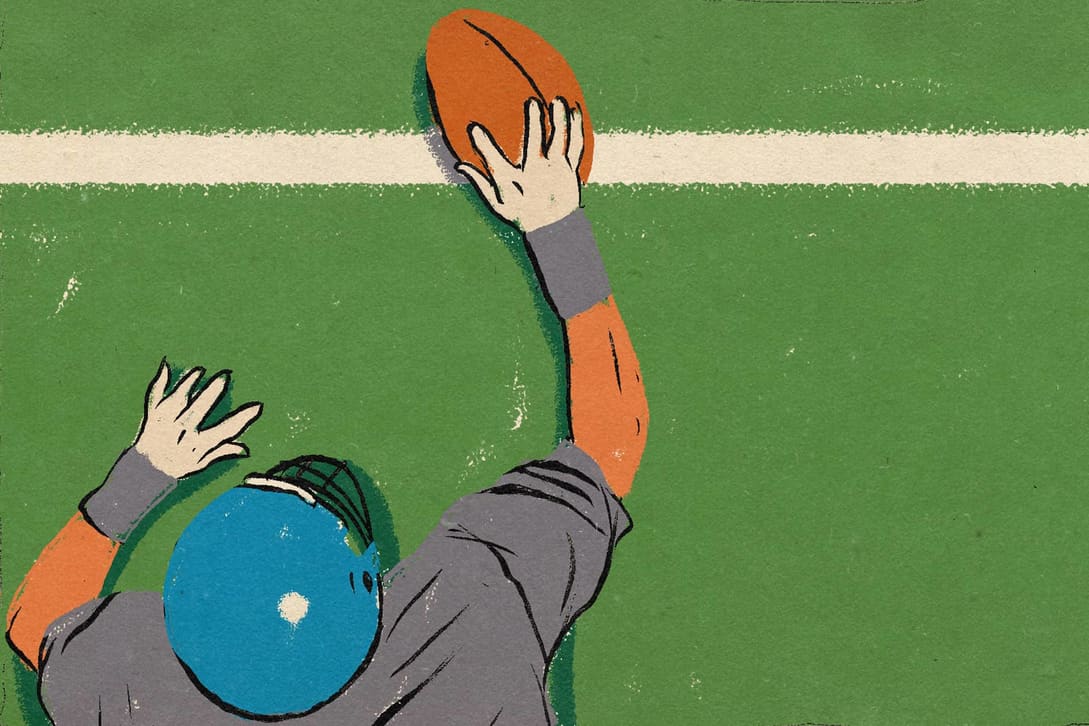This detailed caption synthesizes the essential elements from the three descriptions:

---

This is a vintage-style, cartoon graphic of an American football player from an overhead viewpoint, rendered in a digital clip-art style. The scene captures the moment the player scores a touchdown, with his body laying flat on a green football field textured like paper. The player extends his right arm forward, holding an orange football over a white goal line near the top of the image. 

He's wearing a dark gray jersey with orange sleeves and gray cuffs around his white gloves. Notable are three black horizontal stripes on the back of his jersey and on the sleeve of his right arm. His blue helmet, featuring a face mask and a white spot on top, conceals his facial features. The goal line is a prominent white horizontal stripe, and a long black line runs parallel to it. The football player, positioned in the lower left corner, demonstrates a dynamic pose with both arms outstretched—the right arm higher, decisively planting the football across the goal line to score.